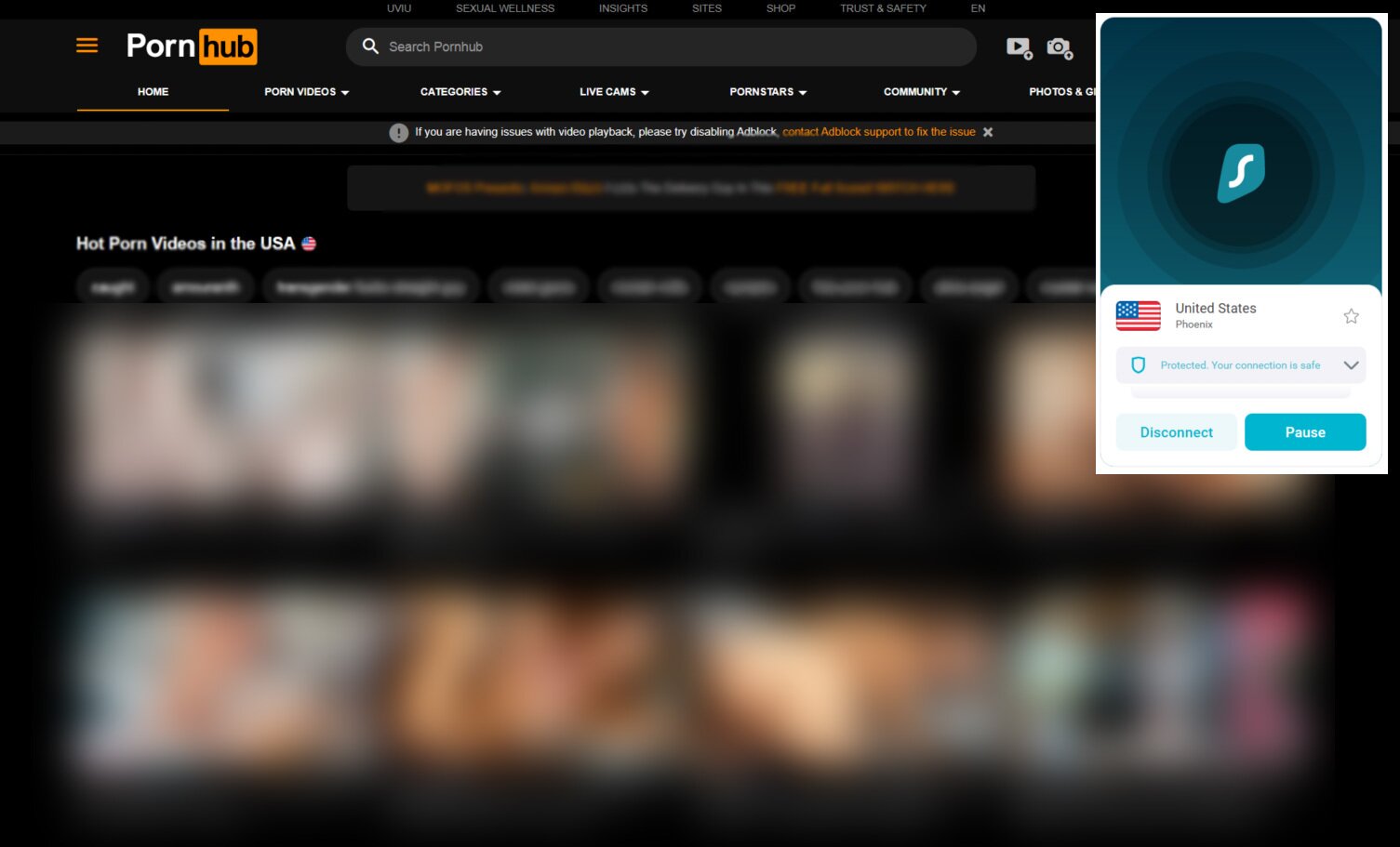The image depicts the top section of the Pornhub website. On the top left, the Pornhub logo is prominently displayed. Adjacent to the logo is a search bar with the placeholder text "Search Pornhub." Beneath the search bar is a navigation menu with the following categories: Home, Porn Videos, Categories, Live Cams, Porn Stars, Community, Photo, and an obscured item. 

To the left of this navigation bar, there is a rectangular tab with a blue background, featuring an icon that resembles a kite. The tab reads "United States," with an unreadable portion below displaying the message "Your connection is safe." Buttons for 'Disconnect' and 'Pause' are also included within this section.

Directly below the navigation menu, a heading reads "Hot Porn Videos in the USA," although the rest of the content and video thumbnails beneath this heading are blurred out. The entire interface is set against a black background.